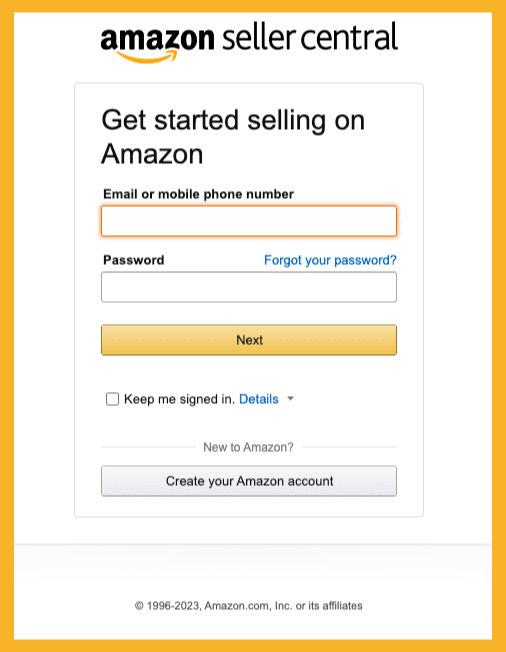The image features an Amazon Seller Central login interface. The framed section has an orange border on the top, right, left, and bottom, enveloping a white interior. At the top is the Amazon logo marked with an orange underline. Below the logo, the text "Amazon Seller Central" is prominently displayed. 

Just beneath, there is a white input box bordered in gray containing the prompt "Get Started Selling on Amazon" in bold black letters. Smaller, fine print underneath invites the user to enter their "email or mobile phone number" with a corresponding white rectangular input box highlighted by an orange border dedicated for user input. Below this, another input box labeled "Password" follows suit, paired with a blue hyperlink on the right reading "Forgot Your Password?"

Completing the form layout, another input box with a gray border awaits the password entry, accompanied by an elongated orange button that reads "Next". Further below, there is an empty checkbox option tagged "Keep me signed in" with a linked "Details" in blue adjacent to it.

Towards the bottom, the interface prompts new users with the message "New to Amazon?" adjacent to a gray button labeled "Create your Amazon account". At the very bottom is the footer text reading "Copyright 1998-2023 Amazon.com, Inc. or its affiliates."